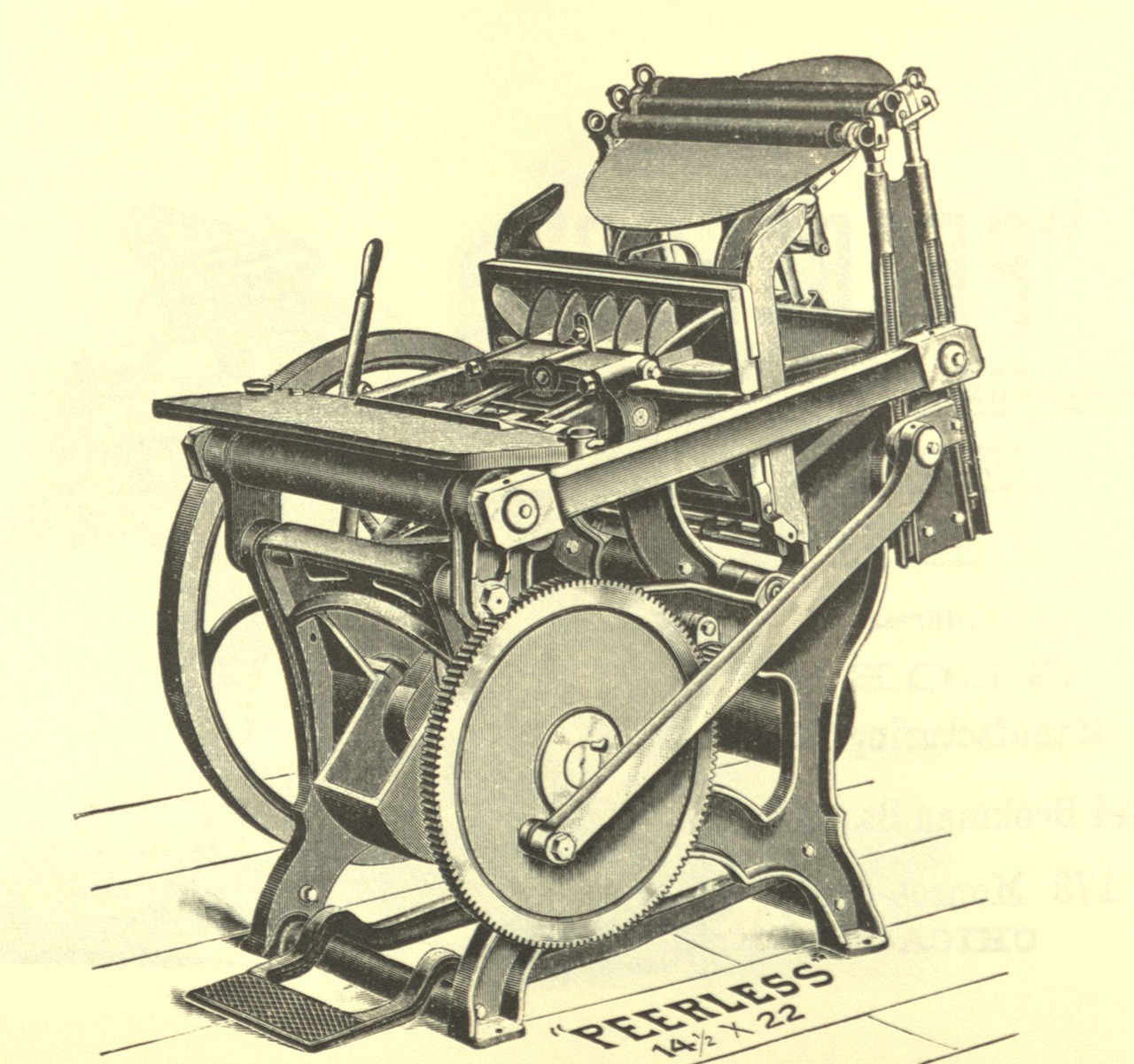This detailed sepia-toned illustration depicts an antique printing press labeled "Peerless 14.5 x 22." The machine is meticulously drawn, showcasing its various mechanical components and intricate design. Positioned on a plank board floor, the printing press features a prominently placed large gear closest to the viewer. A bar extends from this gear, connecting to two vertical arms that lead up to the top of the machine where three rollers are situated above a circular plate. Midway down the press, a square section with blade-like structures is visible, followed by a rectangular platform above another roller. On the right side of the drawing, a large, partially visible turning wheel and several levers are depicted. A foot pedal is located at the base in front of the machine, hinting at its manual operation for the early manufacturing process. The background is a light pink hue, and the machine’s black pencil rendering contrasts starkly against it, emphasizing the detailed craftsmanship of the era.